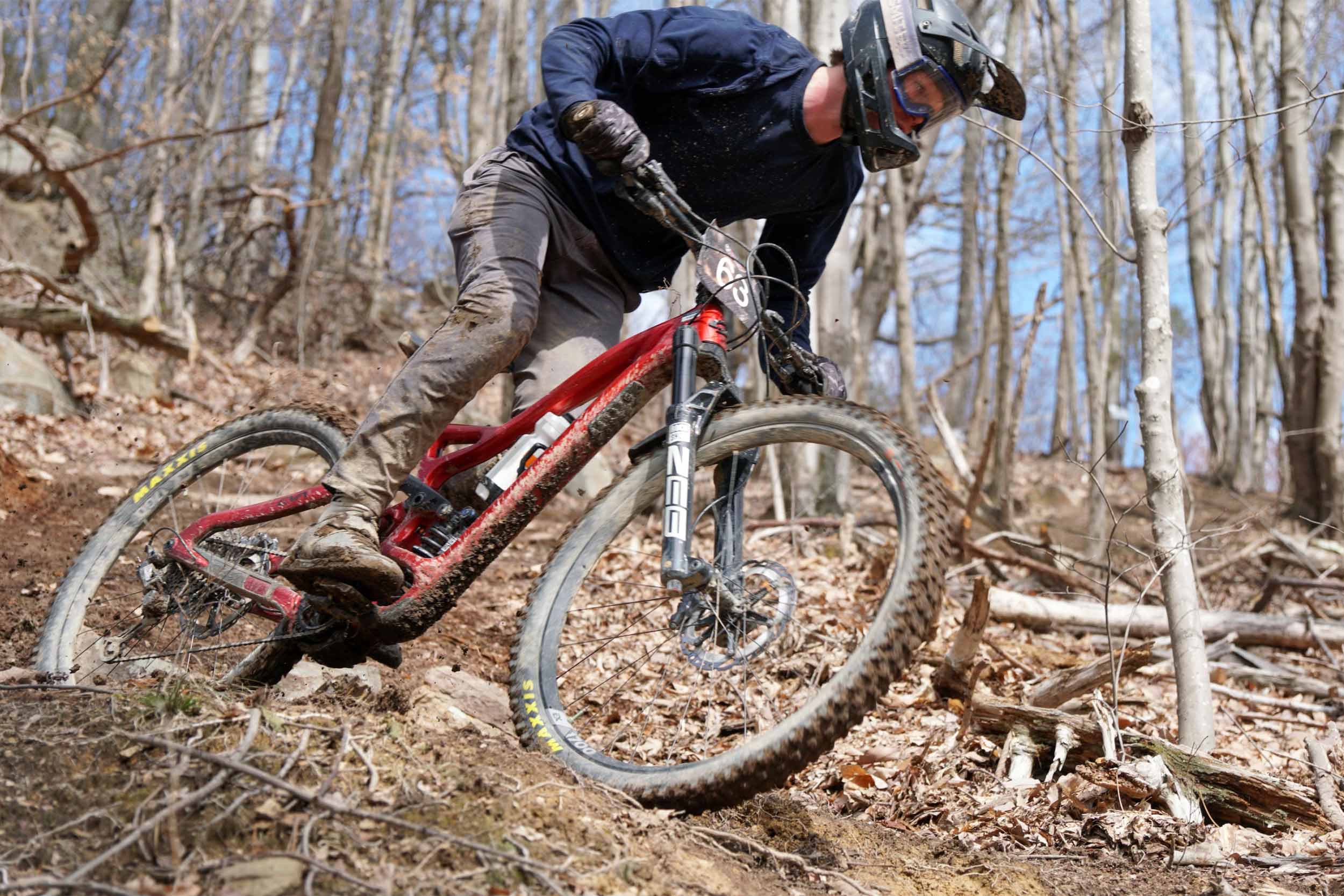The photograph captures a moment during a mountain biking adventure in a dry, dense forest that appears to be in the late summer or fall. There is a man riding down a steep, dirt-covered hill, distinctly not seated but standing on his bike. The forest around him is filled with brown trees devoid of leaves, indicating a possibly arid season.

Central to the image is a red mountain bike with black side handles marked with some black writing, accompanied by black tires featuring yellow lettering. The rider himself is covered in mud, suggesting previous treacherous terrain. He is dressed in khaki-colored pants, brown boots, and a long-sleeved blue jersey. For protection, he wears black gloves, a silver and black helmet, and goggles. Notably, there is a label on the front of the bike, possibly marked with the number '63' or 'B3'.

The scene is set against a clear, sunny sky, with hints of blue peeking through the black and brown canopy of trees, confirming that it is daytime. The earthy colors and fallen leaves on the ground emphasize the transitional season, painting a vivid picture of an intense and exhilarating mountain biking experience.